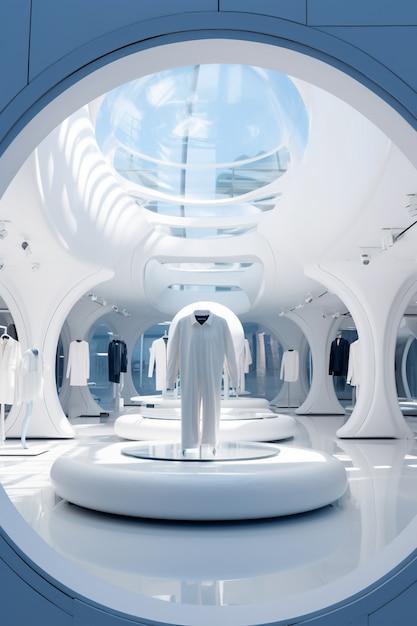The futuristic photograph captures a view through an oval-shaped porthole on what appears to be a spaceship. The porthole, framed with sleek blue metal panels on the top and bottom and bordered by a pristine white rim, provides a window into a modern, all-white room. The room features a shiny, white floor and is supported by minimalist white pillars. Skylights embedded in the ceiling allow natural light to flood the space, enhancing its clean, bright ambiance. Various flat white pedestals are strategically placed around the room, each displaying an assortment of clothing. There are white shirts and pants, as well as standalone white shirts, and even some blue suits, creating an intriguing juxtaposition against the sterile backdrop. The overall scene beams with a sense of futuristic sophistication and minimalistic elegance.